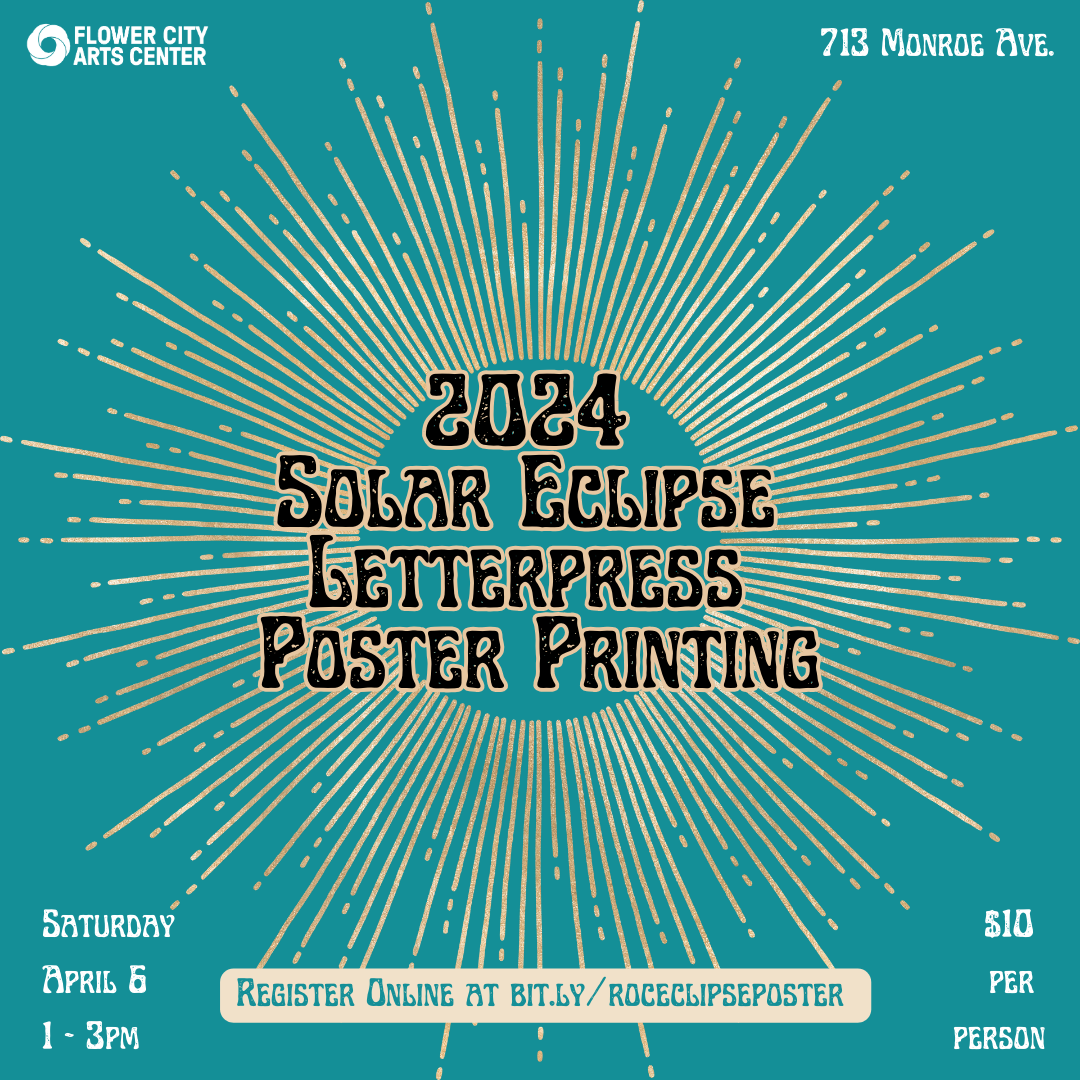The image is a teal-blue poster with a central announcement for the 2024 Solar Eclipse Letterpress Poster Printing event. At the top left corner, the text reads "Flower City Art Center" with an adjacent camera shutter icon, and the top right corner features the address "713 Monroe Avenue." Dominating the center is the event's name, "2024 Solar Eclipse Letterpress Poster Printing," in a distinctive, old-fashioned font. This text is overlaid on a graphic of the sun with radiant sun rays. Below, additional details specify the event date and time as "Saturday, April 6, from 1 to 3 PM." Attendees are instructed to "register online at bit.ly/ROCEclipsePoster," and the participation fee is noted as "$10 per person." The overall design gives an inviting feel, suggesting a family-friendly event centered on creative poster printing.